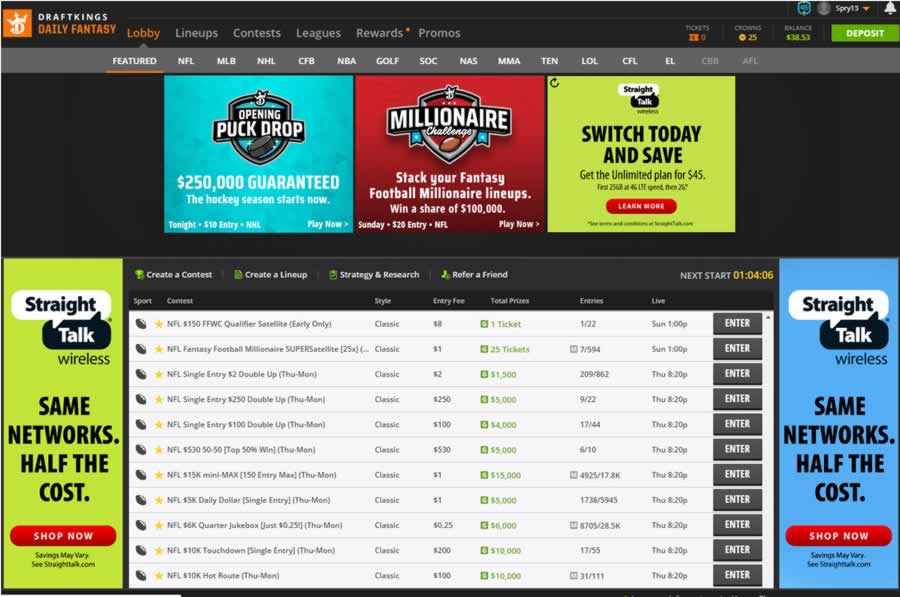**Screenshot of DraftKings Daily Fantasy Platform - Lobby Section**

*In this detailed screenshot of the DraftKings Daily Fantasy platform, we are currently viewing the 'Lobby' section. The navigation bar at the top features several options: Lobby, Lineups, Contests, Leagues, Rewards, and Promos. On the top right, there are icons for Tickets, Crowns, Balance, and a prominent Deposit button. The user’s display name is '513'.*

*The 'Lobby' section provides a variety of sub-options listed horizontally: Featured, NFL, MLB, NHL, CFB, NBA, Golf, SOC, NAS, MMA, TEN, LOL, CFL, EL, CBA, and AFL.*

*Below this, there are promotional banners for various contests and challenges:*

1. **Opening Puck Drop**: A large highlighted square promoting the Hockey Season with a $250,000 guaranteed prize pool. Details include a $10 entry fee and an invitation to play now.
2. **Millionaire Challenge**: This promotional space advertises a fantasy football contest where participants can win a share of $100,000 with a $20 entry fee. The next event is on Sunday.
3. **Straight Talk Ad**: Multiple ads from Straight Talk feature prominently. A central ad promotes saving money with an unlimited plan, detailed as $4.45, $3.25, and $60 at certain levels of service. Additionally, there is a call to action in a red oval indicating an offer to earn more. On the left and right sides of the screenshot are green and blue portrait-style ads from Straight Talk stating “Same networks, half the cost.”

*Central options include buttons for Create a Contest, Create a Lineup, Strategy and Research, and Refer a Friend.*

*Below these options is a grid detailing various NFL contests:*

- **Contest Details**: Each row in the grid elaborates on a specific contest, detailing the sport (NFL), contest type (e.g., $150 FFWC Qualifier, Satellite, Early Only), style (all listed as Classic), entry fee, total prize pool, number of entries, and live start time.

- **Playable Contests**: Examples include:
    - $150 FFWC Qualifier, Satellite, Early Only
    - NFL Fantasy Football Millionaire Super Satellite
    - Single Entry $2 Double Up, $250 Double Up, $100 Double Up
    - Various contests with different entry fees ($530 50-50, $15,000 Mini Max, $5,000 Daily Dollar, $6,000 Quarter Jukebox, and $10,000 Touchdown)
    - Live drawing times are listed (e.g., Next Start: 1 hour, 4 minutes, and 6 seconds).

- **Entry Buttons**: Each contest has an 'Enter' button on the right-hand side, allowing users to participate directly from this screen.

*This screenshot encapsulates a comprehensive view of available contests, promotional banners, and navigation options within the DraftKings Daily Fantasy Lobby, providing users with a seamless interface to engage in fantasy sports betting.*